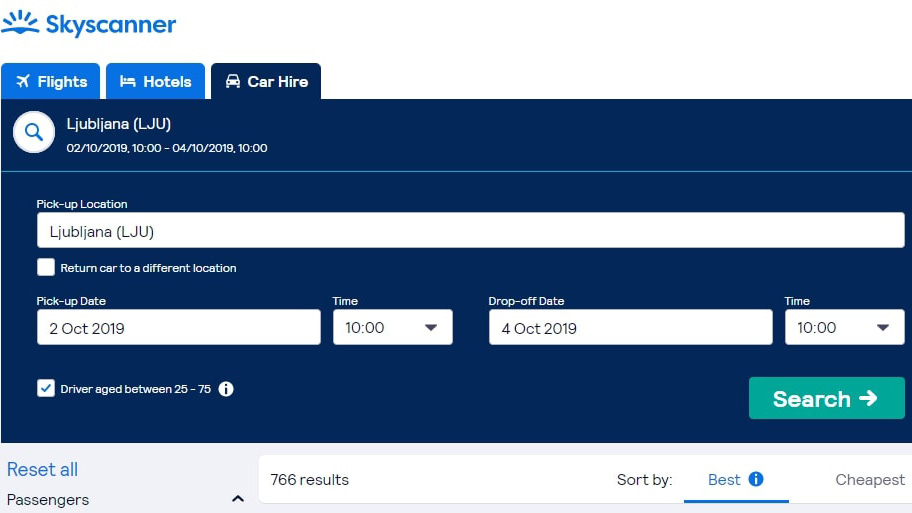Screenshot of the Skyscanner website highlighting its "Car Hire" feature. The website header prominently features the company’s name "Skyscanner" in blue along with a blue icon resembling a sun with rays. The primary background color of the webpage is a dark blue, providing a contrasting visual appeal.

There are three navigational tabs available: "Flights," "Hotels," and "Car Hire." The active tab in the screenshot is "Car Hire," indicated by both its selection and the small car icon adjacent to it. The "Hotels" tab is illustrated with a bed icon, and the "Flights" tab with an airplane icon.

Beneath the tabs, a search interface is displayed with a circular search button. The search is set for car hire in Ljubljana (spelled "L-J-U-B-L-I-J-A-N-A") denoted by the airport code "LJU" in parentheses. The rental period is specified from February 10th, 2019 at 10:00 AM to April 10th, 2019 at 10:00 AM. 

Additional input fields allow users to enter pickup and drop-off details. The pickup location mirrors Ljubljana (LJU). There is an option to return the car to a different location, which is not selected. The specified pickup date and time are October 2nd, 2019 at 10:00 AM, and the drop-off is set for October 4th, 2019 at 10:00 AM. 

This detailed overview captures the core functionality and layout of the Skyscanner Car Hire search interface as shown in the screenshot.